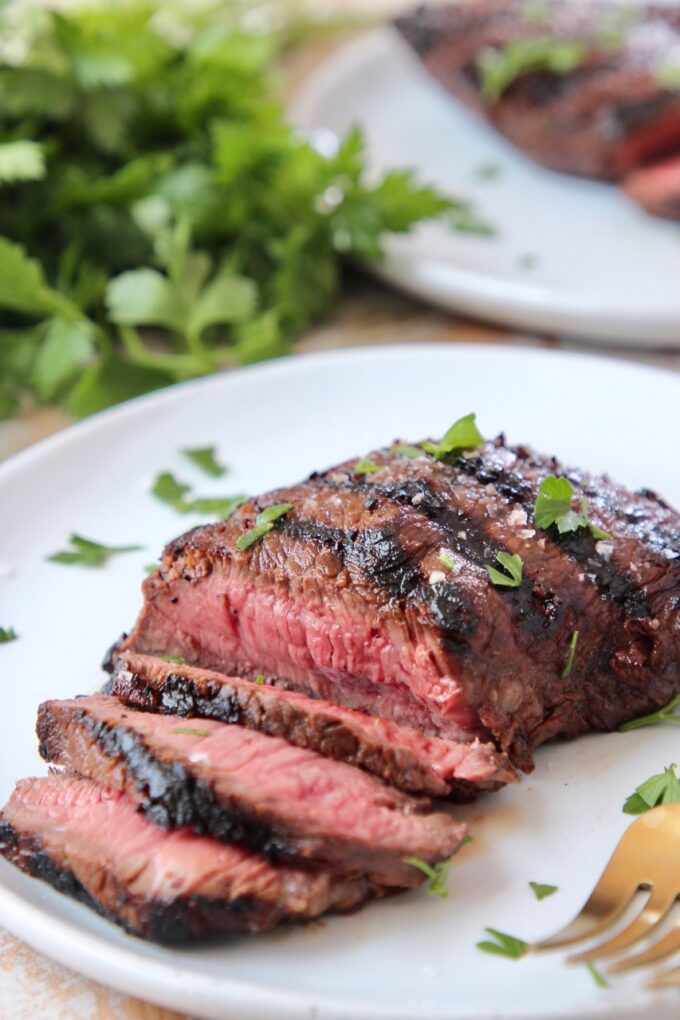The photograph captures a delectable, grilled steak, presented on a large, white ceramic plate. The steak, possibly a filet mignon, is cut into slices, revealing a very rare interior that looks like it might bleed onto the plate when cut. The exterior of the steak is charred with distinct, blackened grill marks, adding to its appetizing allure. Finely chopped parsley, vibrant and fresh, is sprinkled over the top of the steak, adding a touch of green. Toward the right side of the plate, a gold-colored fork points towards the camera, enhancing the composition.

In the background, a bit blurry, is another white plate with more meat and parsley atop it. On the table, which appears to be covered with a brownish tablecloth or wood, rests a bright, fresh bunch of parsley in the upper left corner. The light illuminating this scene is overhead, seemingly from multiple sources, accentuating the rich textures and colors of the dish and creating a warm, inviting atmosphere.